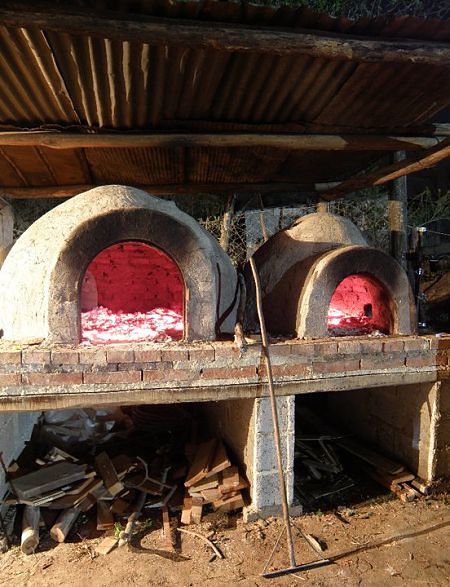The image depicts two dome-shaped, igloo-like clay or brick pizza ovens set in an outdoor pizza restaurant. Sunlight illuminates the front of the ovens, which are suspended on a sturdy structure built from bricks and concrete. Beneath the ovens, there is a storage area filled with wood, likely used to fuel the fires inside. The interiors of the ovens glow with the intense heat of hot coals, casting a red hue, though no pizzas are visible cooking at the moment. A simple wooden roof provides cover several inches above the ovens. The area surrounding the setup features a dirt floor scattered with wood debris and scraps, with some trees visible in the background, enhancing the rustic outdoor ambiance.